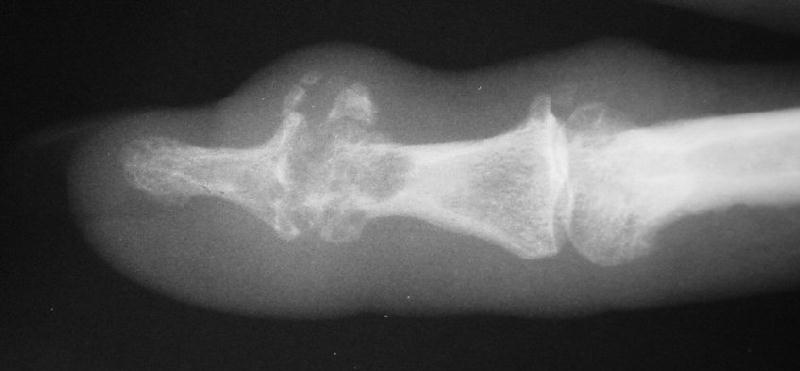This image is a highly zoomed-in x-ray of a section of a limb, most likely a fingertip, prominently featuring black, white, and gray tones. The background is entirely black, drawing attention to the pale white bone in the center. The bone structure includes two smaller bones that connect at a joint near the right-hand side of the image, then taper into a narrow tip towards the left. Around the bones, there is a white aura or gray fog-like smudge, enhancing the bone's outline. The bones appear denser and more opaque near the joint, becoming gradually more translucent as they extend towards the narrower tip to the left. There is no visible text in the image. The overall rectangular shape of the x-ray highlights the intricate details of the bone structure, which may suggest signs of arthritis due to the shape and density variations.